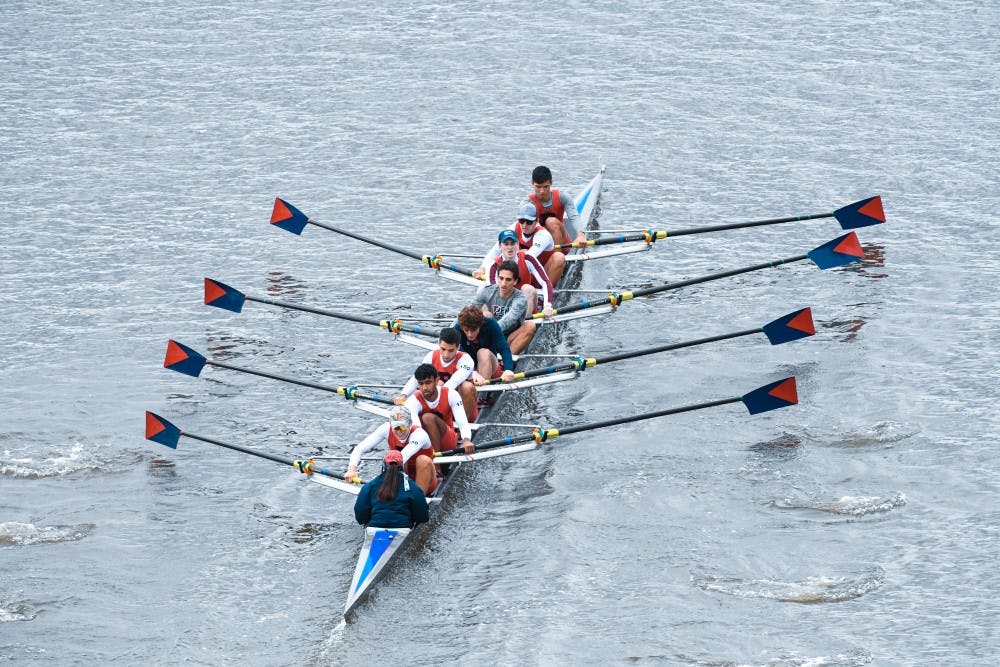The daytime photo captures a group of nine people in a sleek, silver kayak with blue markings at the tip, paddling through water with noticeable currents and white highlights. At the front of the kayak, centrally placed in the image, is an instructor with long hair, wearing a red cap and a blue jacket. Eight rowers are positioned behind, dressed mostly in white long sleeves, red jackets, and red shorts, except for two men in the center, one in a blue sweatshirt and the other in a grey sweatshirt. Each person is holding an oar with alternating sides for paddling, with blue and red paddles. They are moving in unison under the instructor's guidance, showcasing a coordinated effort.